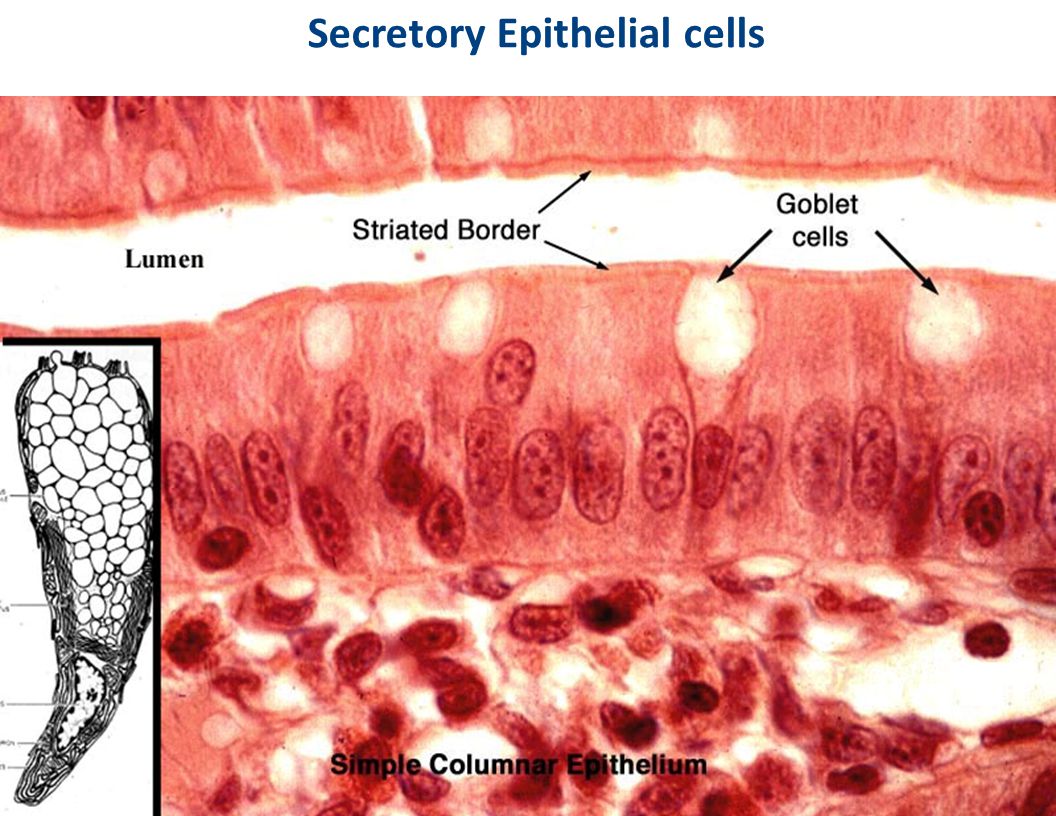The image is a detailed educational slide of Secretory Epithelial Cells, often akin to those found in medical textbooks. The heading at the top, displayed in blue text, reads "Secretory Epithelial Cells." Below the heading is a high-definition microscopic photograph of cellular structures, distinguished primarily with red and white coloring.

The topmost part of the image features a reddish area, representing a layer labeled "lumen," which signifies an internal cavity of a tubular structure. Adjacent to this, in black text, is the label "striated border" with arrows pointing upwards to the lumen and downwards to the next layer. Following this, to the right, the label "goblet cells" is situated, with its corresponding arrow directing downwards towards the white circles depicted within the pink layer below the striated border.

Beneath the goblet cells, a broader reddish area suggests a dense population of cells. At the very bottom of the image, centered black text reads "Simple Columnar Epithelium," indicating the type of epithelial cells shown.

In the bottom left corner, there is a cutout section of the diagram displaying an enlarged view of a different structure. This cutout has a prominent black outline and is filled with pebble-like shapes, likely indicative of another cellular part or structure. The cutout features numbers, though only the number five is partially visible, hinting at a labeled diagram but without further descriptive text.

Overall, this detailed and meticulously labeled image serves as a comprehensive reference for understanding the structure and layout of Secretory Epithelial Cells.